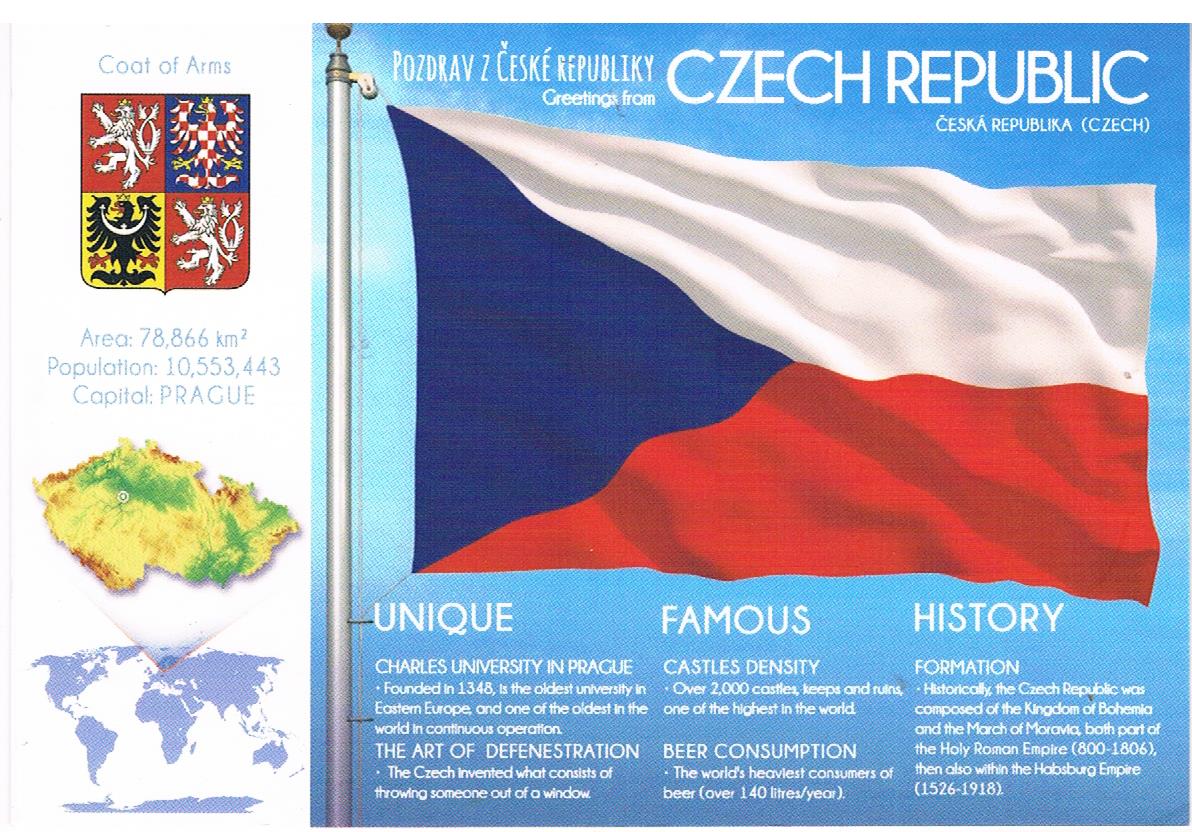This rectangular infographic about the Czech Republic is divided into two main sections. On the left side, positioned within a white column, there are several pieces of information such as the coat of arms, which is depicted at the top in gray text. The coat of arms consists of four square shapes that feature various animals, colored in red, blue, yellow, and black. Following this, the infographic provides key metrics about the country: an area of 78,866 square kilometers, a population of 10,553,443, and the capital, Prague. Beneath these details are two maps, one showing the geographical location of the Czech Republic and another a zoomed-in world map.

On the right side, the background is a vibrant sky blue, enhanced with an image of the Czech Republic's flag. The flag features a white and red rectangle intersected by a dark blue triangle on the left, shown hanging from a silver flagpole. At the top right, large white text reads "Czech Republic," with smaller white text above it saying "greetings from." Beneath the flag, the infographic is divided into three categories of information: unique, famous, and historical.

In the unique section, the infographic highlights Charles University in Prague, founded in 1348, noted as the oldest university in Eastern Europe and one of the oldest in the world with continuous operation. The famous section lists the Czech art of defenestration, the country's high density of castles, with over 2,000 castles, keeps, and ruins, and mentions their prominent beer consumption, over 140 liters per year, making them the world's heaviest consumers of beer. The historical section explains the formation of the Czech Republic, detailing its historical composition of the Kingdom of Bohemia and the March of Moravia, both part of the Holy Roman Empire from 800 to 1806, and later within the Habsburg Empire from 1526 to 1918.